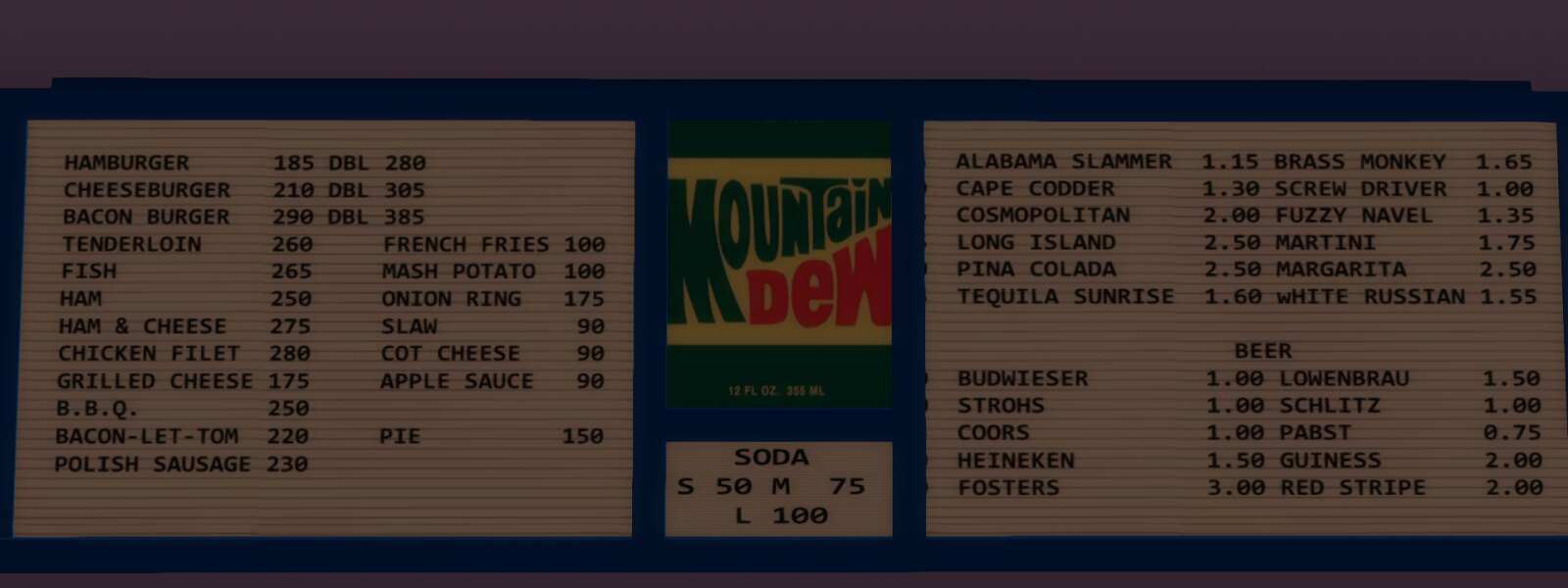This dimly lit color photograph captures the nostalgic interior of a vintage restaurant, primarily focusing on a large white menu sign that dominates the image. The menu features a prominent, classic Mountain Dew logo in the center, with "Mountain" fully spelled out, indicating the photograph likely dates back to the late 1970s or early 1980s.

Below the logo, various soda sizes and their prices are displayed: a small soda is priced at $0.50, a medium at $0.75, and a large at $1.00, further emphasizing the era's affordability. The left side of the menu lists a variety of food items under low prices, such as a hamburger for $1.85. The listed items include a range of offerings from hamburgers, cheeseburgers, and bacon burgers to tenderloin, fish, ham, ham and cheese, chicken filet, grilled cheese, barbecue, BLT, and Polish sausage.

On the right side of the menu, a selection of drinks is featured, including mixed cocktails like Alabama Slammer, Cape Codder, Cosmopolitan, Long Island, Piña Colada, and Tequila Sunrise, each priced very affordably, with the Tequila Sunrise costing only $1. Additional cocktails such as Brass Monkey, Screwdriver, and Fuzzy Navel are also listed. 

Furthermore, the menu includes a variety of beers, featuring brands like Budweiser, Stroh's, Coors, Heineken, Foster's, Guinness, and Red Stripe. The nostalgic atmosphere evoked by the menu’s pricing and selection provides a charming glimpse into a bygone era of dining.